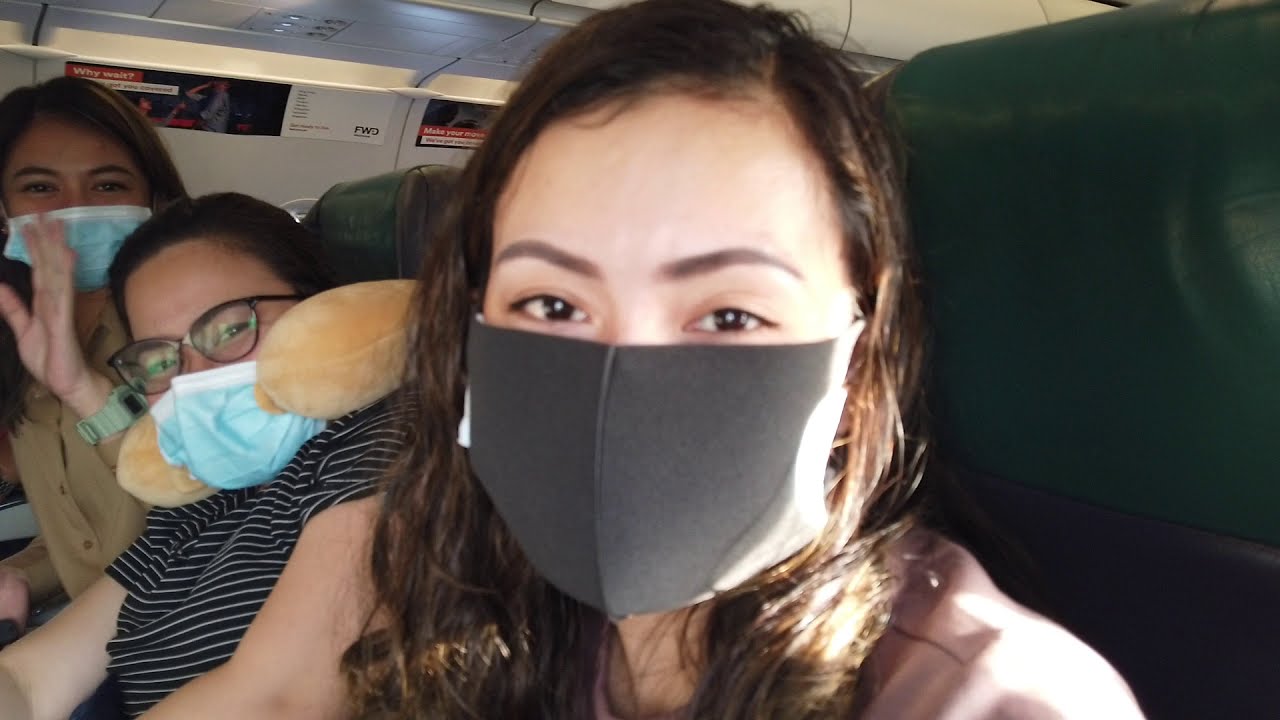The photograph shows three happy girls on an airplane with green seats, all smiling under their face masks. The girl in front has brown hair and wears a black face mask, while the one behind her, with black hair and glasses, dons a blue mask and a light brown neck pillow. The third girl, also with brown hair and a blue mask, sports a green watch on her left wrist. In the background, the airplane's overhead compartments display banners with the text "why wait" and more visible wording. Their happiness is evident, even though their smiles are hidden by their masks.